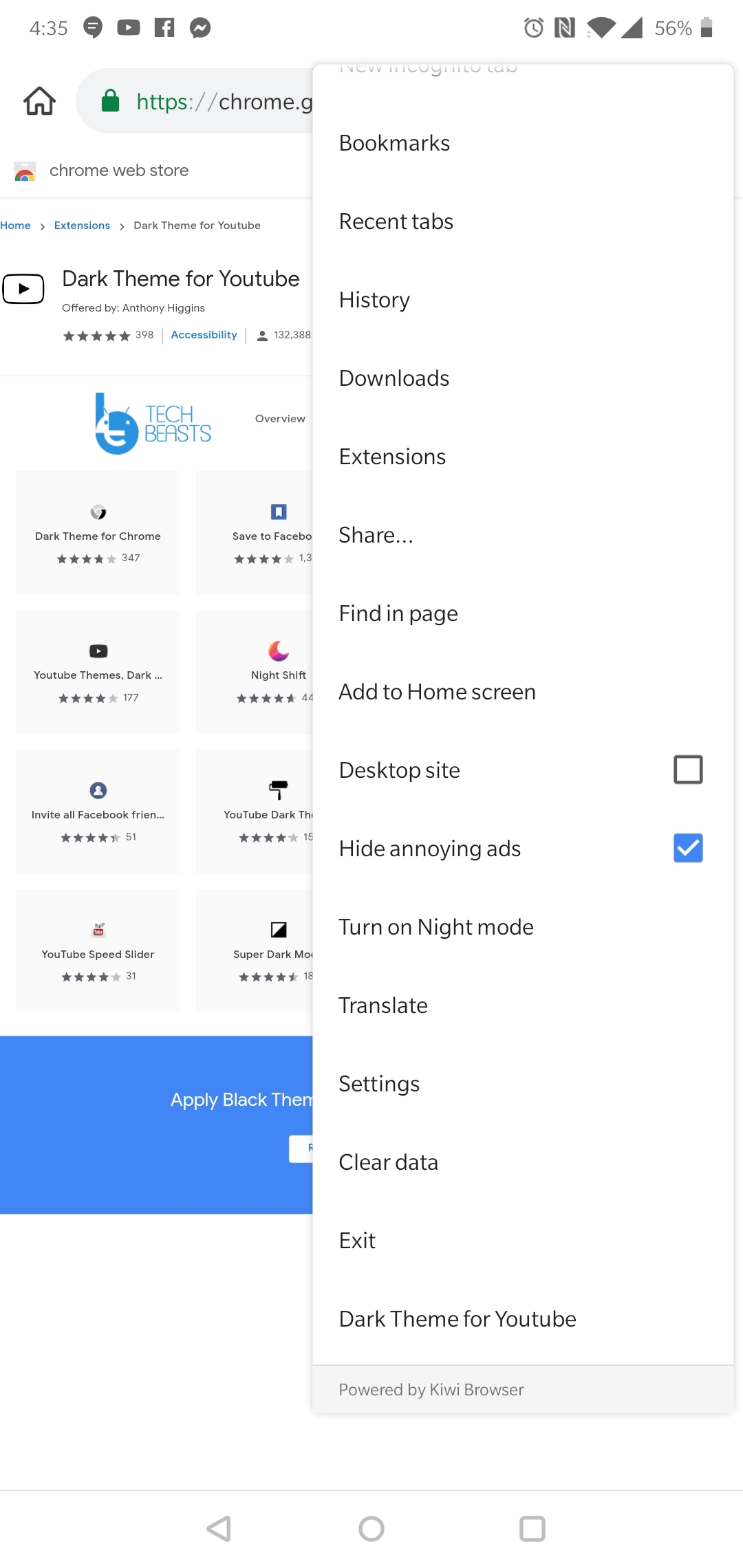A person is browsing the Google Chrome Web Store on their smartphone. The screen shows the left half of the Chrome Web Store interface and a settings menu on the right. The settings menu is extended, covering a significant portion of the right half of the display. In the background, the main page features a "Dark Theme for YouTube" app along with several similar apps aimed at providing dark themes for various services like YouTube and Chrome. These apps are presumably designed to alter the usual interface color to black or dark blue.

The extended settings menu lists numerous options including bookmarks, recent tabs, history, downloads, extensions, share, find in page, add to home screen, desktop site toggle, hide annoying ads (which is currently enabled), turn on night mode, translate, settings, clear data, and exit. It also shows that the "Dark Theme for YouTube" has already been installed, allowing the user to enable or disable it from this menu.